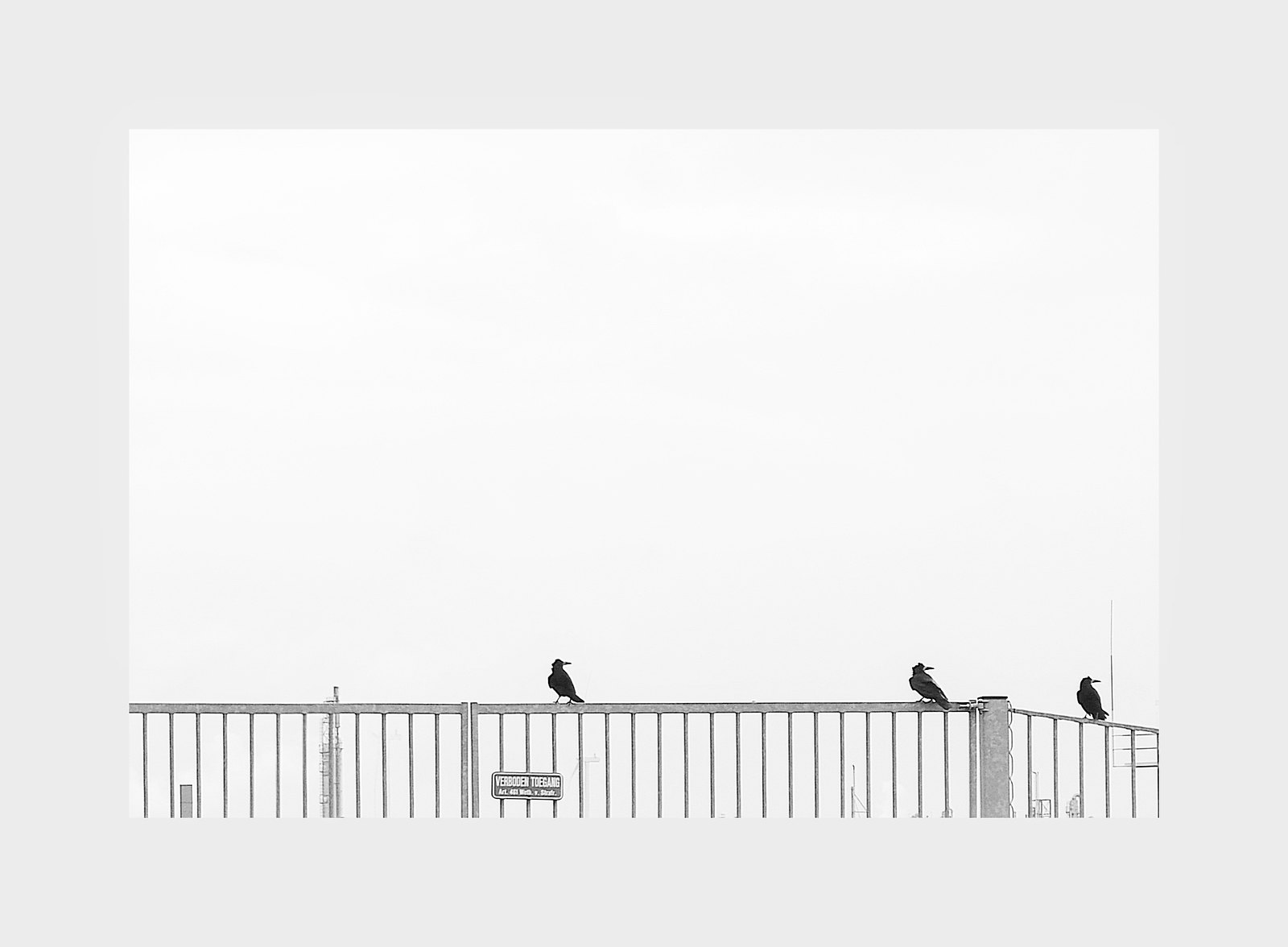This image displays an animated sketch of three black crows perched on the top rail of a gray fence. The crows, all seen from a backside and slightly elevated viewpoint, are attentively looking to the right into the distance. The fence features a central post, creating the impression of observing a corner section, with continuous light gray lines extending downward beneath the rail. The scene is enveloped by a predominantly white background with subtle gray undertones, suggesting a cloudy or foggy urban setting. There's also a small, unreadable sign attached to the fence rail. Overall, the birds are spaced apart along the rail, adding to the stillness and contemplative feel of the artwork.